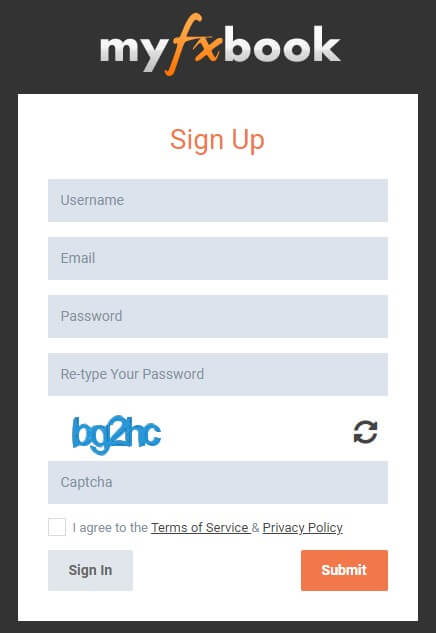The image depicts a registration page for "myFXbook," characterized by its distinctive color scheme and layout. The header "myFXbook" features the word "my" in white, "FX" in orange, and "book" in white, set against a black background that frames the entire image, occupying the top 10-15% of the space. The background below the header is predominantly white.

Directly beneath the header, a red "Sign Up" prompt is visible. Below this prompt, four gray rectangular fields are arranged vertically, labeled sequentially as "Username," "Email," "Password," and "Retype Your Password." Further down, a patch of code marked "BG2HC" in blue is placed alongside a refresh icon.

Following these elements is another gray rectangle labeled "CAPTCHA," accompanied by a checkbox stating "I agree to the terms of service and privacy policy." In the lower section of the image, on the left side, a gray rectangular button reads "Sign In," while on the right, an orange button with white text instructs "Submit."